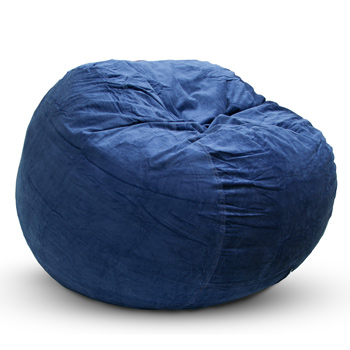This image captures a large, navy blue bean bag chair set against a completely white background, likely indicative of a studio photo shoot. The bean bag, made from a suede-like textured fabric, has a round, somewhat spherical shape with the top being slightly pressed in and wrinkled, suggesting recent use. A shadow is cast on the smooth white floor beneath it due to the overhead lighting, which also highlights the varying shades of blue on the chair, making it appear slightly darker at the bottom. The bean bag is notably full and leans a bit to the left, with the back side raised slightly. Overall, the image is clean, detailed, and meticulously captured to highlight the product.